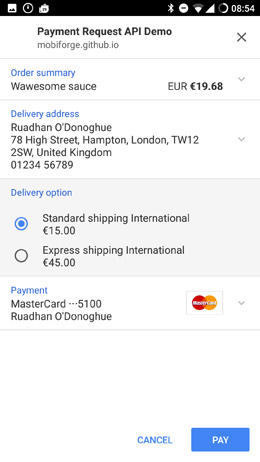The image appears to be a screenshot taken on a mobile device. At the top of the screen, there is a thin black banner with three indistinct icons on the left and multiple icons on the right, including Bluetooth, a circle symbol, the cellular strength indicator, the Wi-Fi strength indicator, an additional small symbol, and the current time.

Beneath this banner, the screen features a white background segmented by thin gray lines into distinct rows. 

- **First Row:** Bold text reading "Payment Request API Demo," followed by "MobiFord.github.io" underneath, and an 'X' icon to the right.
- **Second Row:** On the left, blue text that says "Order Summary," followed by "Wasmsauce" below it. To the right, it displays "EUR" plus the Euro symbol (€) and the amount in bold: "€1968." There is a drop-down button beside this information.
- **Third Row:** Contains "Delivery Address" in blue text. Below this, a London address is listed for a person named Wuodan O'Donoghue.
- **Fourth Row:** A gray box titled "Delivery Options" with selectable choices. Currently, "Standard Shipping International" is selected, costing "€15." Additionally, there is an option for "Express Shipping International" for "€45," although it’s not shown in full.
- **Final Row:** On the left, blue text indicating "Payment." Underneath, it shows "MasterCard ...5100" and further down, the cardholder's name. To the right, there's the MasterCard logo and another drop-down button.

Each element is clearly set apart, making the information easy to digest at a glance.